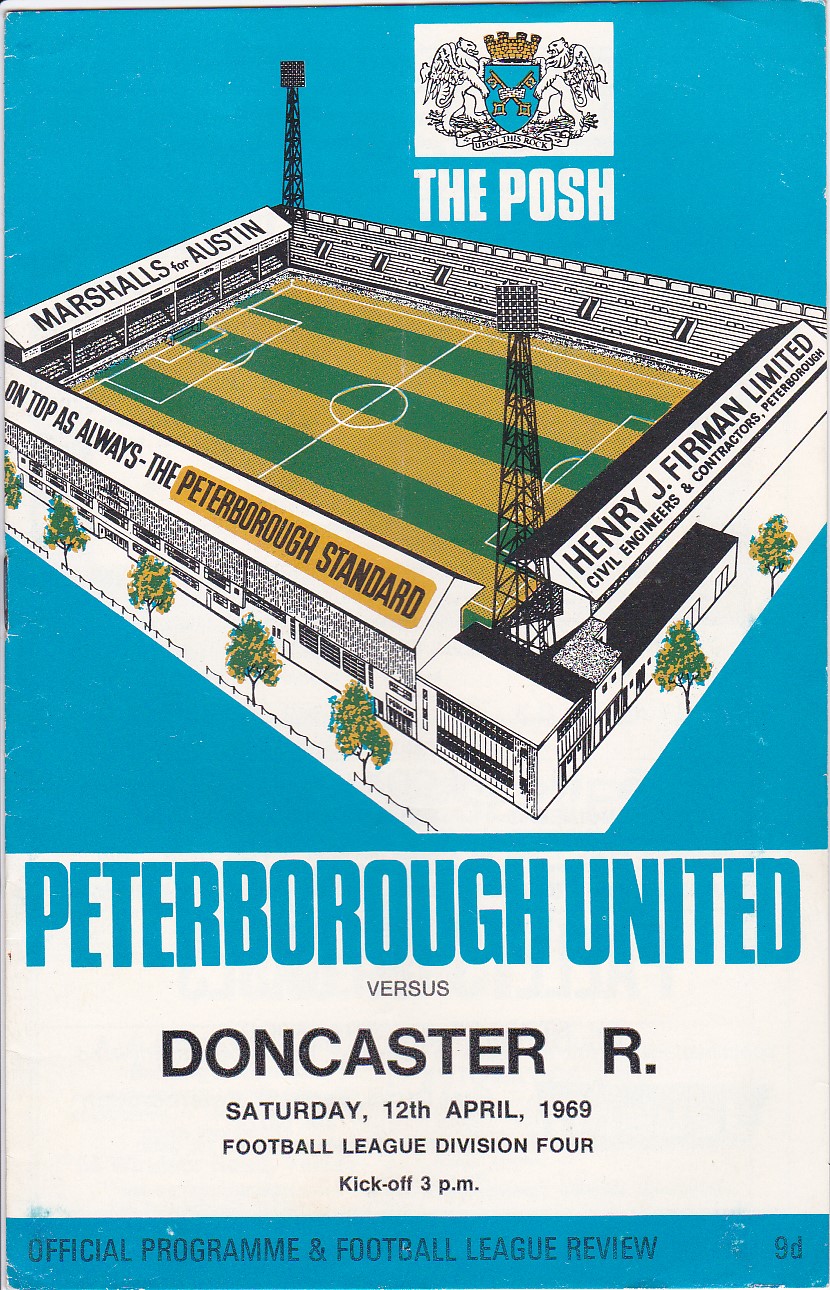The image depicts the cover of an official program for a soccer match. The background is a light blue with a detailed illustration of a stadium at the center. The field is visually striking, composed of alternating yellow and green stripes with white lines marking the boundaries and areas typical of a soccer pitch. Surrounding the field are stands with black and white seating areas.

At the top of the cover is an ornate emblem featuring two griffins holding a blue shield adorned with a gold crown. Beneath this emblem, in white text, it reads "The Posh." Flanking the stadium illustration are advertisements in black text: on the left side, "Marshalls and Austin," and on the right side, "Henry J. Furman Limited, Civil Engineers and Contractors."

Below the image of the stadium, on a white background, the details of the soccer match are presented in light blue and black text. It announces "Peterborough United" and underneath, in smaller black text, "versus Doncaster R." Below that, the date "Saturday, April 12, 1969," the event "Football League Division IV," and the kickoff time "3 p.m." are listed. The bottom of the program notes it as the "Official Program and Football League Review 9-D" in a black text on a light blue section.